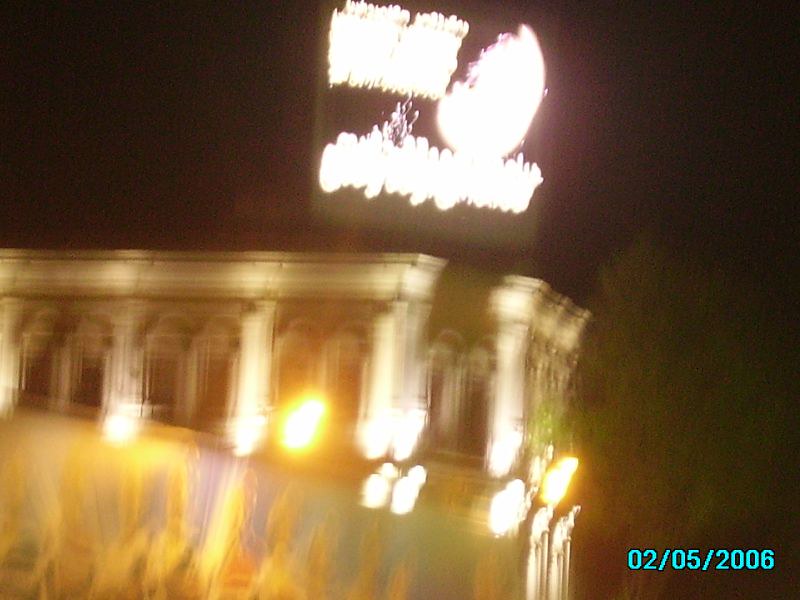This blurred photograph, dated 02-05-2006 in blue writing at the bottom right corner, captures a nighttime scene of a grey building with prominent white columns and arches. The top of the image features a black screen displaying bright lights in the shape of two rectangles with a circular object in between. Just beneath this are multiple bright lights illuminating parts of the building's façade. The midsection of the structure showcases white and yellow lighting, and below the arches, there appear to be windows, though they are not clearly visible. A distinctive gold and purple painting partially covers the building. In the foreground, yellow grass-like plants are discernible, and on the right-hand side, a green tree or bush stands out. The dark sky provides a stark contrast, highlighting the building’s illuminated architectural features.